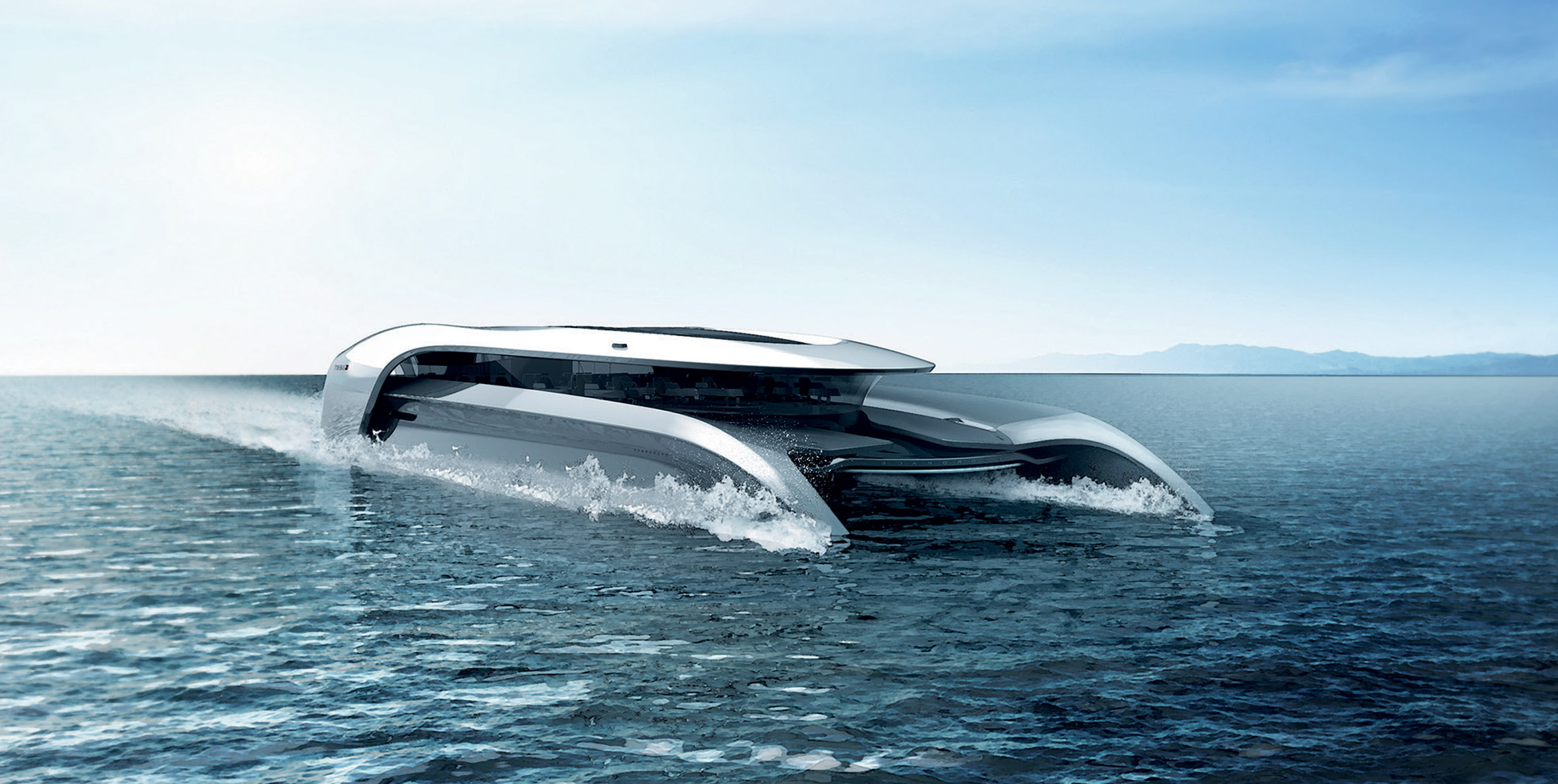In this color photograph, an ultramodern, sleek, metallic silver boat glides through the dark, opaque, greenish-blue waters of the ocean. The vessel, resembling an extraterrestrial aircraft, is distinctive with its angular, platinum features and curved design that seamlessly maneuvers through the water, leaving a wake behind it. The scene is predominantly muted and dull, with a mostly white sky containing hints of blue and light cloud cover, creating a grayish atmosphere. In the distance, indistinct shapes suggest the presence of a tree line, hills, or mountains, adding depth to the composition. There are no visible people, animals, or identifiable markings in this image, which focuses exclusively on the interaction between the futuristic boat and its serene, expansive aquatic environment.